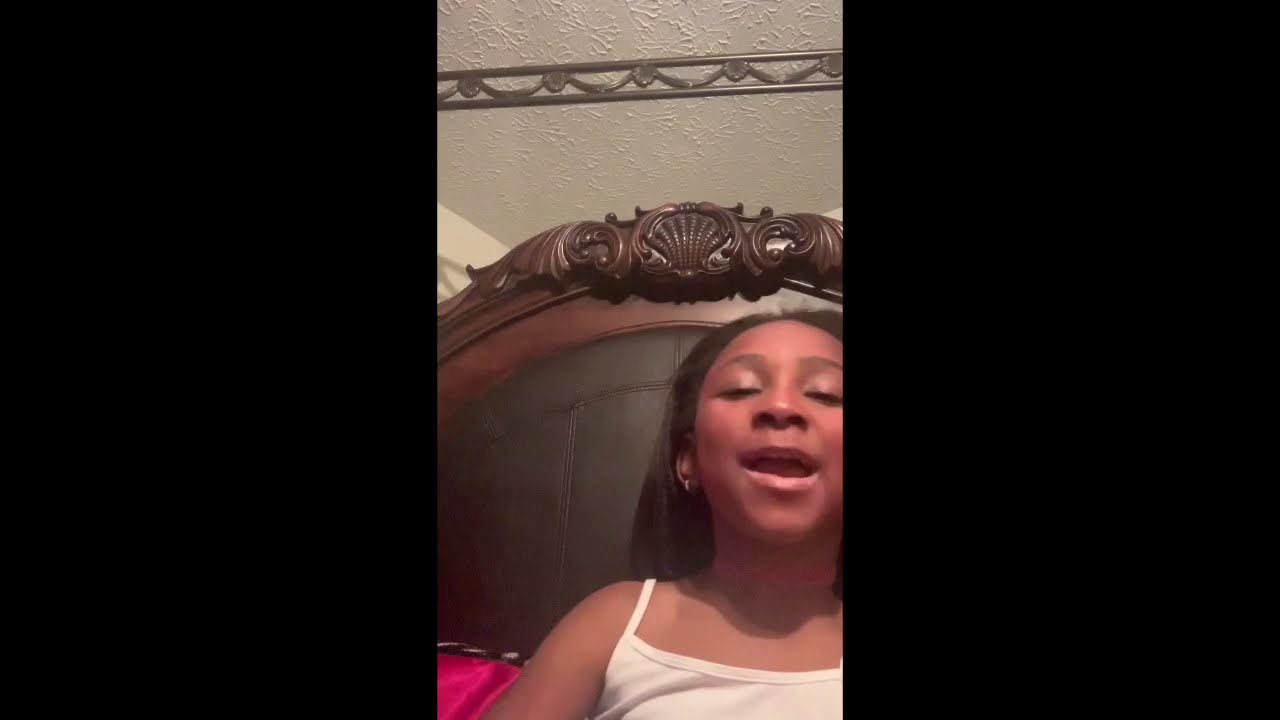In the image, we see a young black girl with shoulder-length black hair, dressed in a white spaghetti strap tank top. She is resting on a bed, positioned against an ornately designed headboard made of dark wood with lighter brown and black edges. The headboard's top features decorative carvings resembling little feather wings on the sides and a central clamshell design. The girl appears happy, with her mouth open as if singing or talking, although her teeth are not visible. Her head is slightly tilted back, and her eyes are mostly closed, possibly adorned with eyeshadow. She is wearing an earring in her left ear. A pink blanket is draped beside her, and the bedding includes a striking red pillow or bed sheets with a black edge. The ceiling above is white, featuring a black bar running just beneath it. The walls are also white, providing a simple backdrop to the scene.